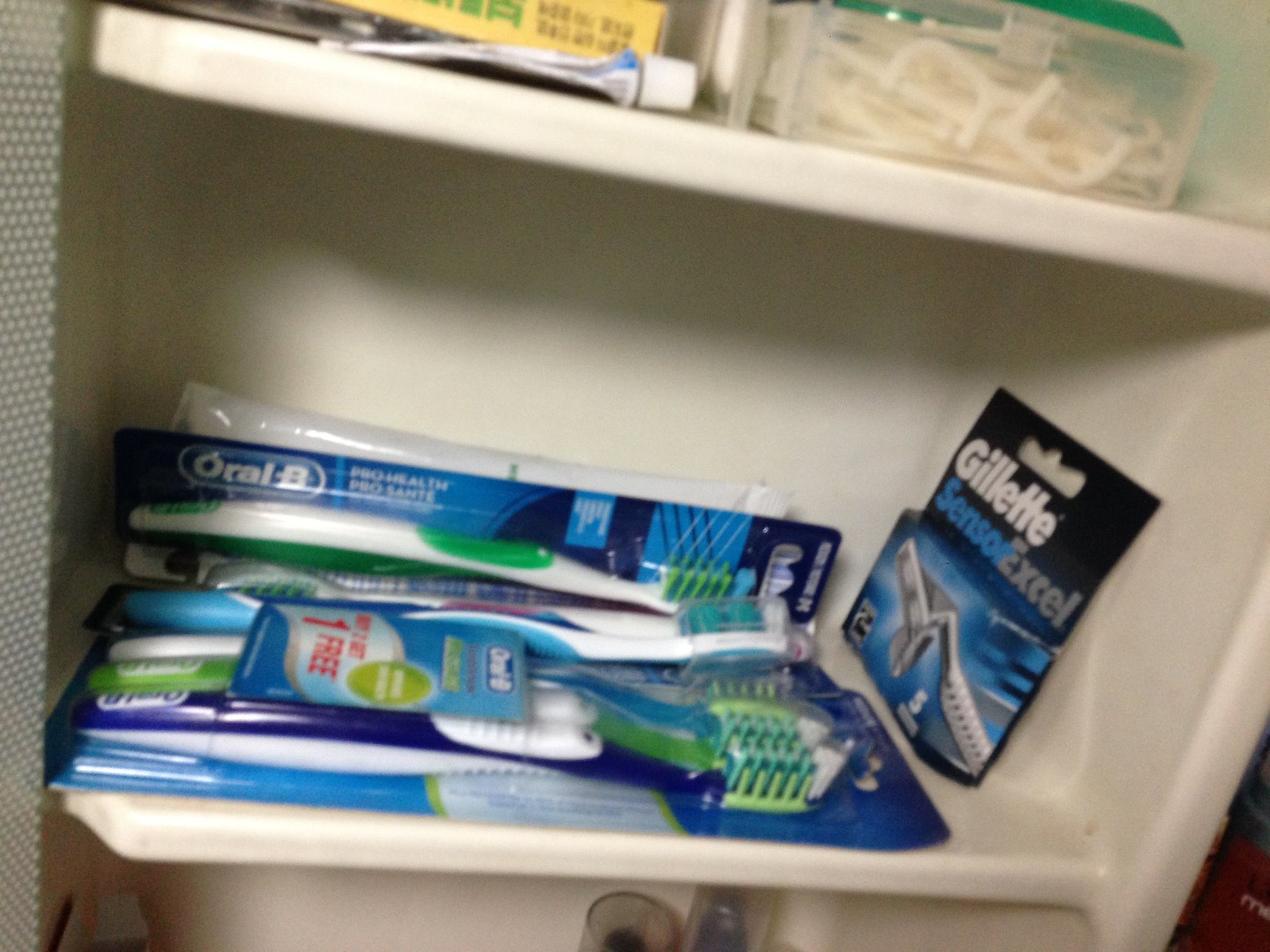This image depicts a white, off-white medicine cabinet, likely located in a bathroom. The cabinet comprises multiple shelves, though not all are fully visible. On the top shelf, partially cut off at the edge of the image, there is a small clear case containing white plastic dental flossers, with an indeterminate green item on top. A partially used tube with a white cap and a yellow box, whose contents are unclear, also occupy this shelf.

The focus is mainly on the middle shelf, which prominently showcases several packages of Oral-B ProHealth toothbrushes, still in their packaging. The toothbrushes feature green, blue, and white handles, and appear to come in multi-packs of three, totaling five or six packages. To the right of these toothbrushes stands a Gillette Sensor Excel razor package, which is blue with white and gray writing and includes a visible picture of the razor on the front, indicating it’s a five-pack. Additional items on the middle shelf include more Oral-B toothbrush packages, again characterized by their green and blue color schemes.

The lower part of the cabinet is slightly visible, yet it’s challenging to discern specific items there. The clean, organized setup of the cabinet underscores a focus on dental hygiene products, specifically toothbrushes, flossers, and razors.